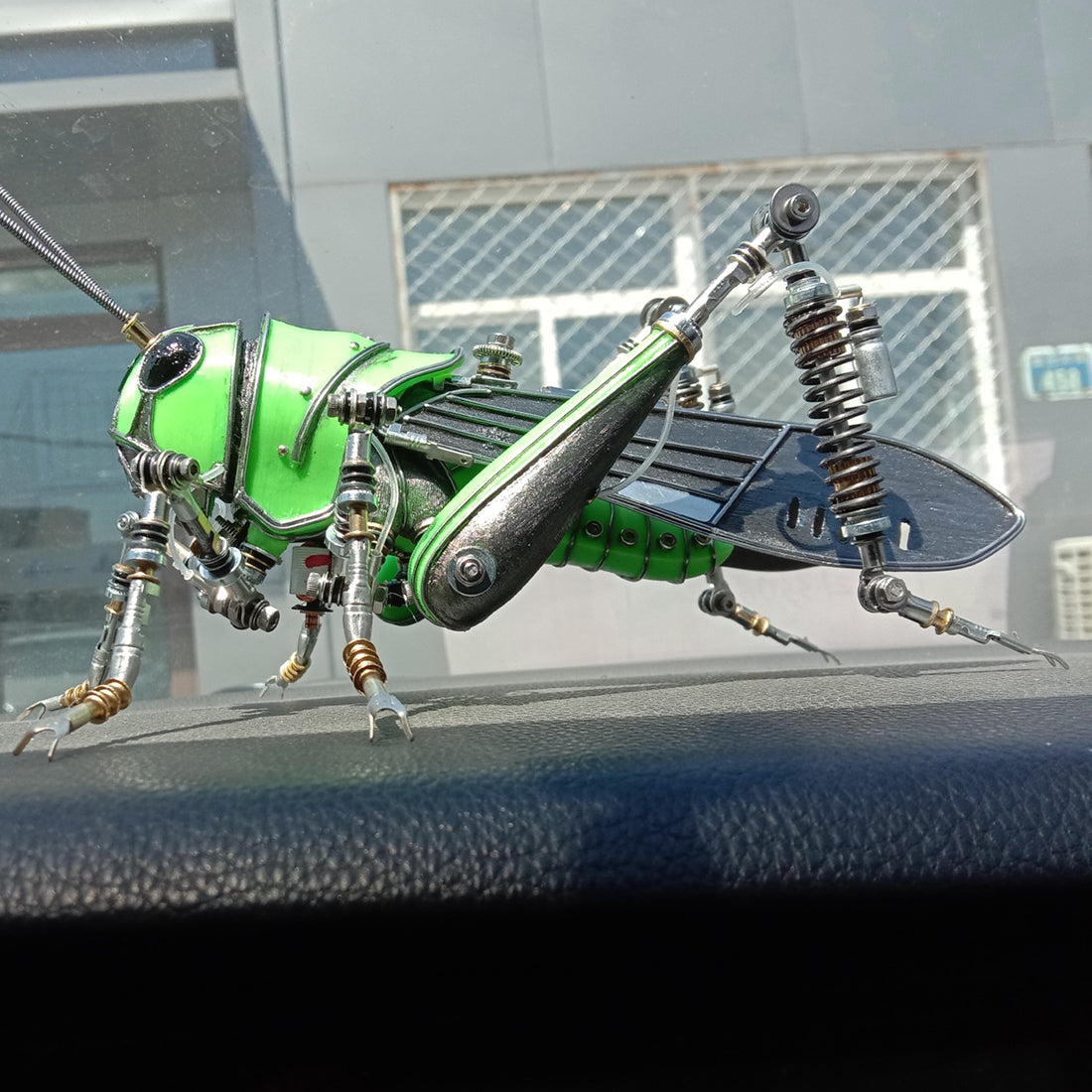The photograph features a detailed metal sculpture of an insect, modeled intricately to resemble a grasshopper or possibly a cricket-like robot. The sculpture boasts a lime green body with shiny black eyes and metal components, including six elaborately designed legs with spring-like mechanisms suggestive of hydraulic or suspension systems. The front legs have two claws each, while the back legs are equipped with shock absorber-like springs. Two metal antennae extend from its head. The grasshopper is positioned on a leather-like surface, likely the dashboard of a car. In the background, part of a building is visible, along with some window reflections, hinting that the photo was possibly taken inside a vehicle. The composition appears to be unprofessional, suggesting the image was captured with a smartphone. The intricate details and artistic nature of the sculpture strongly suggest that it is a piece of art intended for aesthetic appreciation.